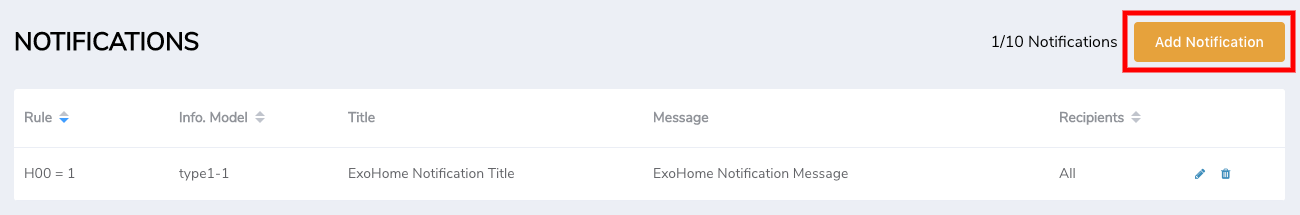The image displays a notification management interface on a light gray background with dark gray or black text. The header, located on the left side, prominently reads "Notifications." On the right side of this header, it indicates "1 of 10 notifications," suggesting the user is viewing the first of ten notifications.

On the extreme right side, there is an orange button with white text that reads "Add Notification." This button is highlighted with a red outlined box, drawing attention to its functionality.

Below the header, a table is presented with several columns labeled: Rules, Info Model, Title, Message, and Recipients. Each column contains respective information for notifications. The initial entry in the table includes the following details:
- **Rules:** H00 equals one
- **Info Model:** Type 1-1
- **Title:** XO home notification title
- **Message:** XO home notification message
- **Recipients:** All

Additionally, there are small icon buttons for editing or deleting the notification, represented by a pencil and a trash can icon respectively. These icons are minimalistic and positioned next to the notification entry.

The image appears to be cropped, focusing narrowly on this section of the screen. Its purpose seems to be instructional, possibly showing users how to add a new notification, as indicated by the circled "Add Notification" button. The overall design suggests it might be a demo or template screen for guiding users through the notification adding process.